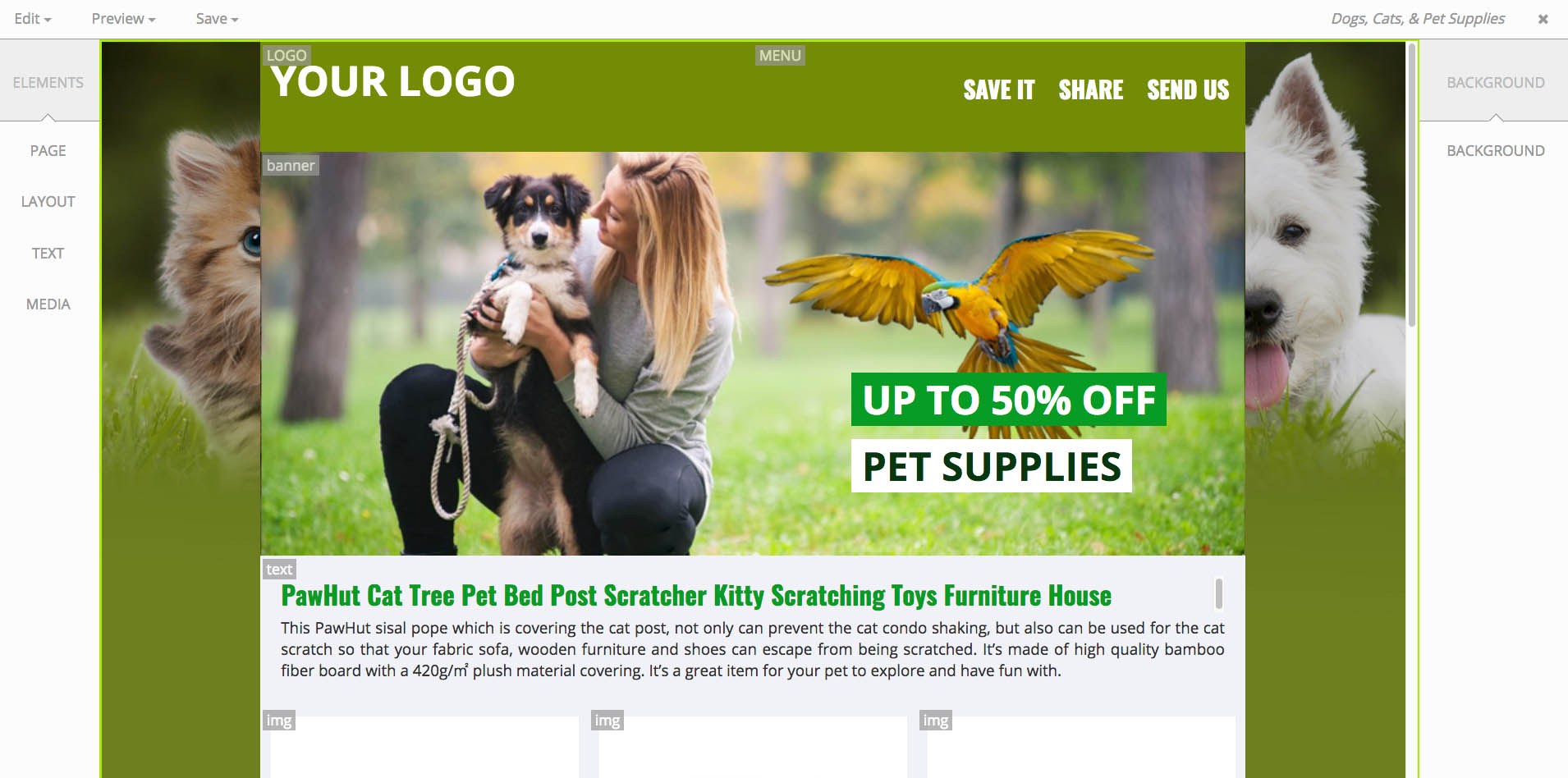This is a detailed screenshot of a sample website under development. At the top, a light grey navigation bar spans across the screen. On the top left corner of this bar, there are three drop-down buttons labeled "Edit," "Preview," and "Save." On the right side of the same grey bar, a search field displays the text "dogs, cats, and pet supplies" with an "X" button beside it. 

To the left of the screen is a vertical sidebar featuring five tabs labeled "Elements," "Page," "Layout," "Text," and "Media."

In the main content area, a green horizontal bar stretches across the top, showcasing the website's logo prominently in white text on the left. On the right side of this bar, there are additional options labeled "Save," "Share," and "Send Us," all in white text.

Below the green bar, a large photo banner highlights a woman crouching down while holding a brown and white dog with floppy ears. This banner spans the page, providing a welcoming visual element to the site.